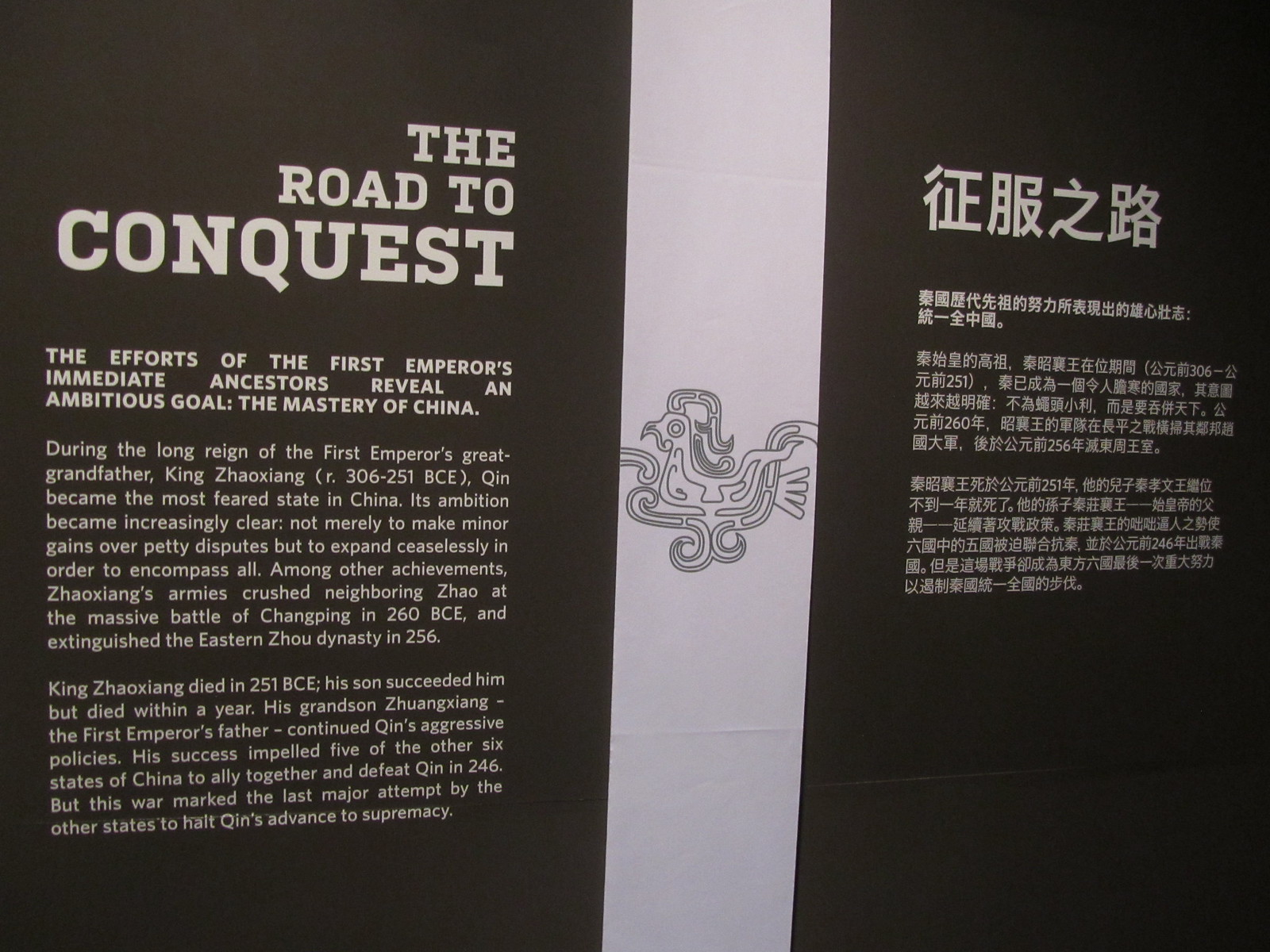The image features two black signs placed side-by-side against a dark background. The sign on the left is in English, while the one on the right is in Chinese. Between these two signs, a narrow off-white vertical strip runs down the middle, featuring a simplistic, black-and-white sketch of a bird facing left. The bird drawing appears somewhat cartoonish and is rendered in a primitive, pencil-like style.

On the left sign, the text begins with a bold title that reads "The Road to Conquest." Beneath this, it states, "The Efforts of the First Emperor's Immediate Ancestors Reveal an Ambitious Goal: The Mastery of China." Following this introduction, two paragraphs detail specific historical figures, focusing on King Zhaoxiang, discussing his long reign and significant contributions. The right sign, entirely in Chinese, likely mirrors the information presented in the English text.